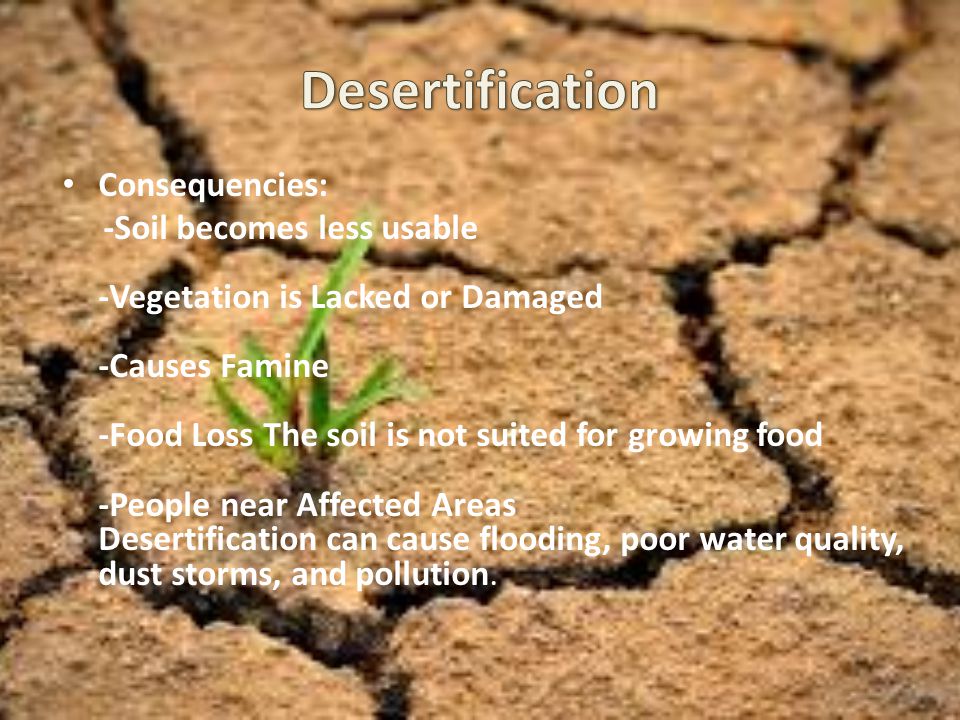The image depicts parched, cracked earth reminiscent of severe drought conditions with no moisture. At the center-left of the barren landscape, a singular small sprig of grass emerges, symbolizing a fragile beacon of life in a devastated environment. Overlaying the image is prominently displayed white text. At the top center, the capitalized title "Desertification" sets the theme. Below it, a section labeled "Consequences:" lists several bullet points: "Soil becomes less usable," "Vegetation is lacked or damaged," "Causes famine," "Food loss," "The soil is not suited for growing food," and mentions that "People near affected areas" experience dire impacts. Additionally, desertification can lead to "Flooding, poor water quality, dust storms, and pollution." The overall layout of the text suggests it resembles a PowerPoint slideshow presentation.